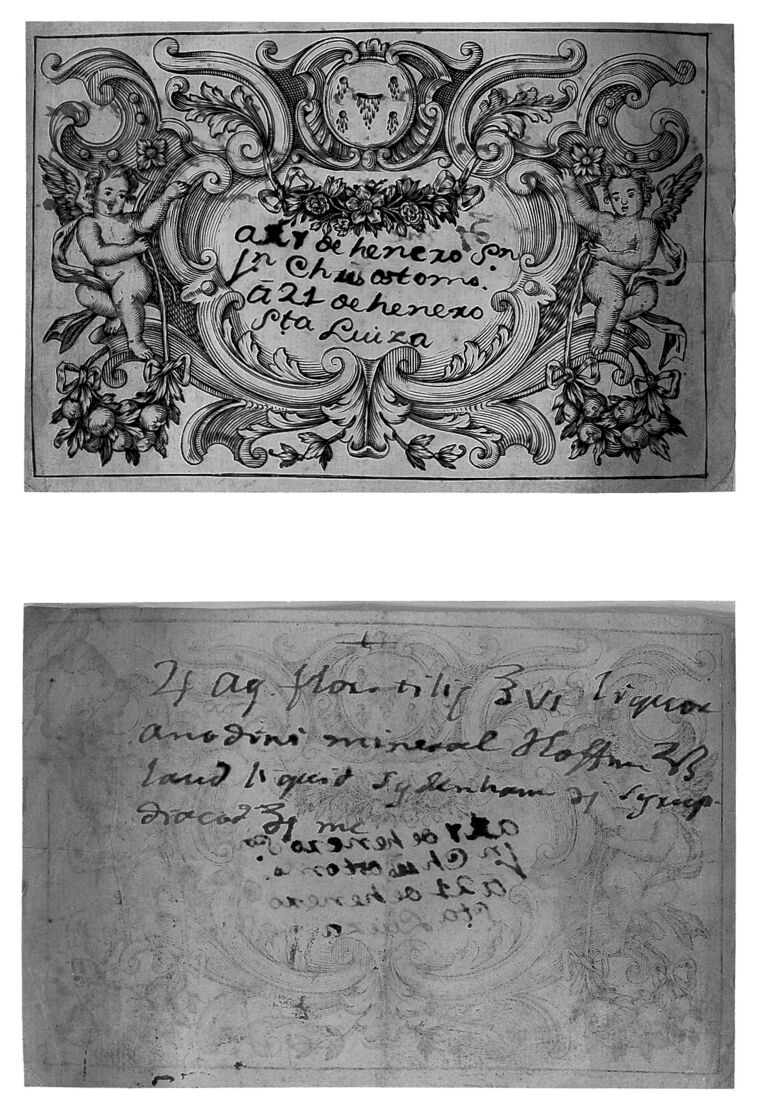The image depicts both the front and back of a grayscale postcard that seems to be from several years ago. The front side features intricate, hand-drawn designs reminiscent of the ornate flourishes seen on dollar bills. Dominating the top center of the card is an emblem or crest, vaguely resembling a Ouija board, inscribed with the letters "S-T-A-L-U-I-Z-A." Flanking this central motif are two cherubic figures—one on the left, one on the right—each with wings and curly hair, seemingly interacting with an elaborate floral arrangement and possibly holding harps. The postcard's border is adorned with additional delicate, swirling patterns. The back of the postcard contains handwritten script, likely in a non-English language, scrawled hastily in black ink, suggesting it might be a message to the recipient. Overall, the image exudes an air of antiquity and artistic detail.